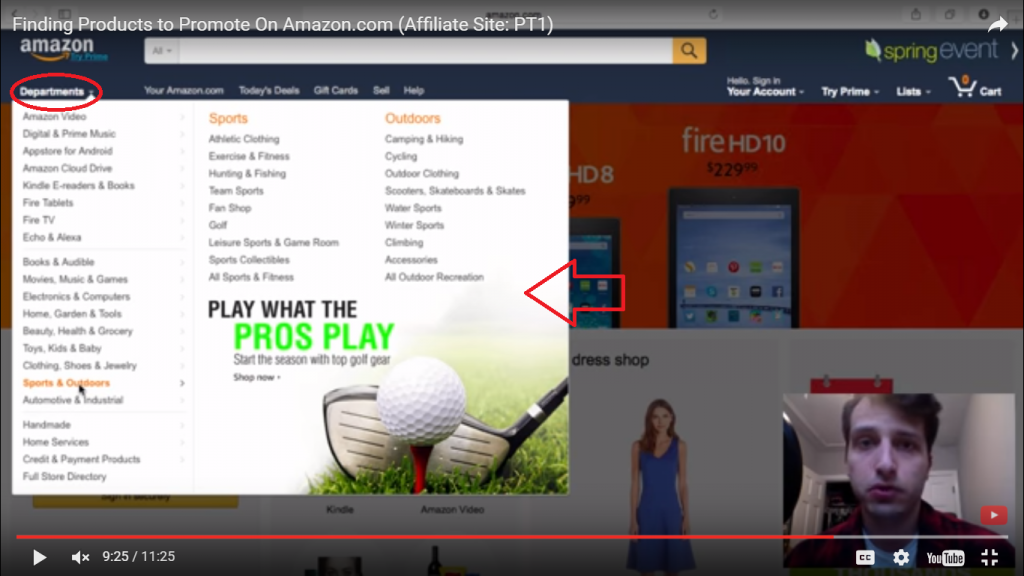In this image, we observe a detailed screenshot of the Amazon.com homepage. The site showcases a variety of features and categories. At the top, there's a sign-in option for personal accounts, followed by a list of core services including a shopping cart and a highlight of the current "Spring Event." To the left, a navigation pane displays an extensive list of departments such as Amazon Video, Digital Music, Store for Android, Amazon Cloud Drive, and Kindle e-readers. It also includes categories for books, Fire tablets, TV, movies, music, games, electronics, computers, home, garden, tools, clothing, grocery, toys, and more. Additionally, specific sections for children’s and baby clothing, shoes, jewelry, sports, outdoors, home services, and other utilities are present. Furthermore, there are specialized areas for athletic clothing, exercise and fitness equipment, hunting gear, professional sporting gear, top golf gear, and canine paraphernalia.

Toward the bottom, the image focuses on the Fire HD 10 tablet. Adjacent to this, there’s a prominently featured image of a person looking directly at the camera, suggesting a product demonstration or promotional video. Notably, the video section includes controls for volume and display, highlighting that the video is muted and currently at 9 minutes and 25 seconds of a total 11 minutes and 25 seconds, with options for full screen and YouTube capture.